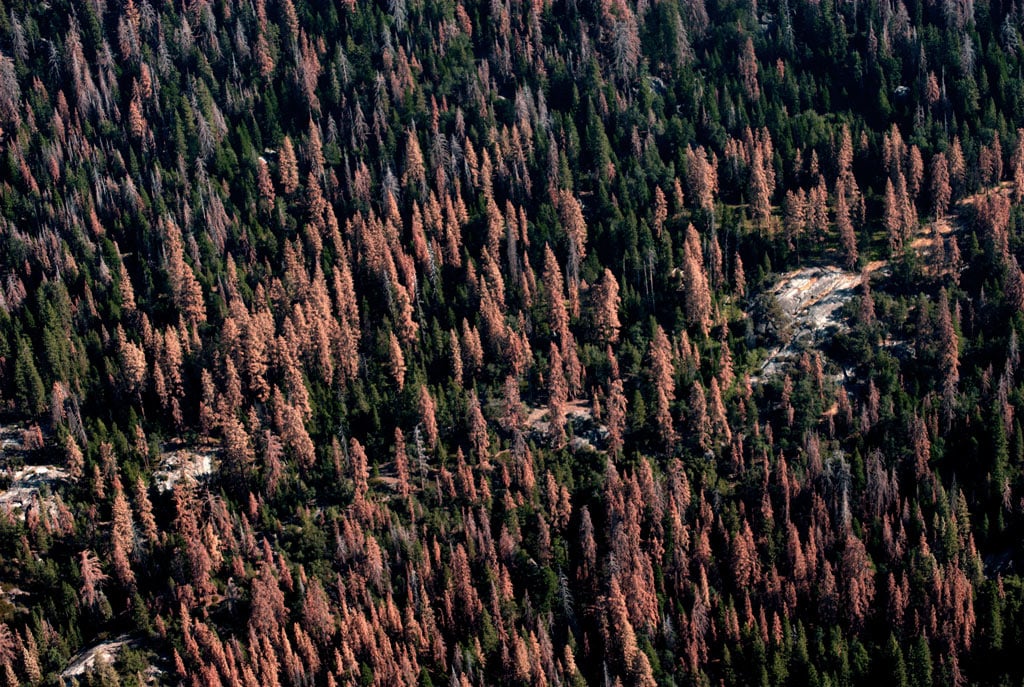This aerial image, likely taken from an airplane or drone, showcases a dense forest. The forest is a vibrant mix of green and pink-hued trees, creating a colorful scene that stands out under the sunlight. Cutting through the middle of the forest is a distinct, white, icy path, either a river or creek, adding an intriguing element to the landscape. The view is so high up that the trees appear small, further reinforcing the vastness of the densely packed forest. Additionally, some areas suggest a possible serpentine shape or line of snow weaving through the vegetation, amplifying the mystique of this nature-filled image.